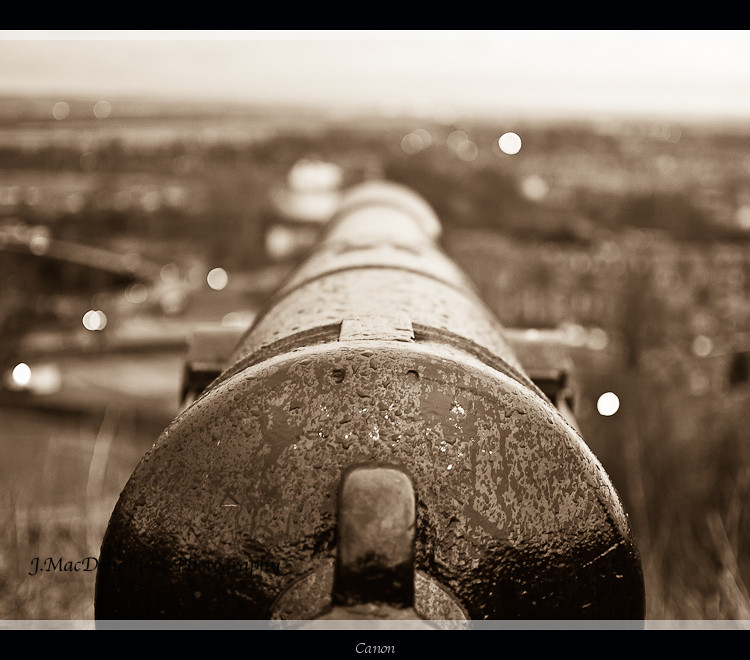This black-and-white photograph depicts a 19th-century cannon, taken from directly behind and looking down the length of the barrel. The perspective suggests the photographer stood behind the cannon, aiming straight over its elongated barrel towards a distant cityscape that is blurred but identifiable through the faint outlines of small buildings. The only part of the image in sharp focus is the rear of the cannon, which is speckled with water droplets, indicating it was likely taken after a rain or during a moment of early morning dew. At the bottom of the picture, a black border displays the white word "CANNON," although a misspelling is noted with one 'N' missing. Additionally, the signature "J. MacD..." appears on the left side of the image, partially obscured by the dark shadow of the cannon. The overall composition, including the cannon's gleaming wet surface and the hazy background, gives the photograph a historical and almost somber atmosphere, potentially reminiscent of a monument in Cranford, New Jersey.